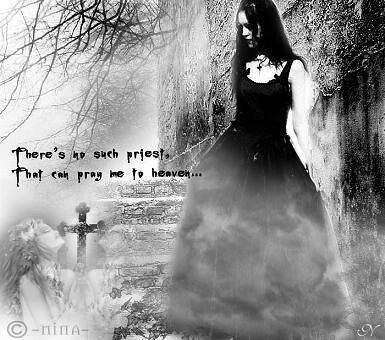The black and white image, reminiscent of an album cover, features a solitary woman in a solid black dress with medium-length black hair, walking down a stone staircase in a foggy courtyard, cemetery, or garden area. She is adorned with a cross necklace and stands amidst a backdrop of old, spindly, and dying trees. The environment is heavily shrouded in mist and evokes a somber, eerie mood. At the bottom left of the image, a slightly obscured figure of another woman with closed eyes appears to be on the ground, looking upward. In this corner, the text "©-Nina-" is stamped. The focal point of the image is a towering cross to the left of the woman, accompanied by the haunting, drippy-font inscription above it: "There's no such priest that can pray me to heaven..." To the right, intertwined with the fog at the bottom of the dress and overall atmosphere, mysterious tree limbs and shrubbery add to the ghostly, unsettling aesthetic.